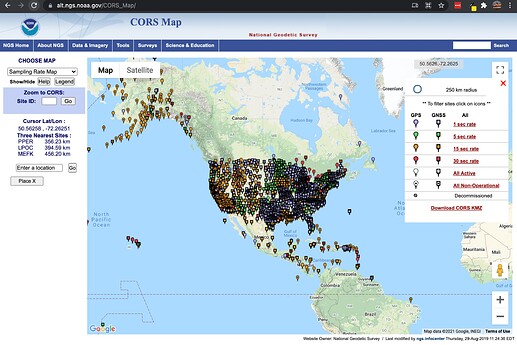The image depicts a detailed CORS map from a website with a light blue strip across the top. In the center of this strip, it reads 'CORS Map' in standard text. Prominently displayed in red font across the top is the title 'National Geodetic Survey.' On the left side of the screen, a small section marked ‘Choose Map’ offers various options, although the text is tiny and difficult to decipher. The available map types seem to include options like 'Survey Rating Map' or 'Rain Map.'

Below this, a small blue box contains input fields labeled 'Set ID' and 'Zoom in CORS,' accompanied by dynamic data showing the cursor’s current latitude and longitude coordinates. This box also lists the three nearest geodetic survey sites.

The primary map itself spans from Brazil to the Arctic Circle in northern Canada, featuring a stark contrast of pin densities and colors. Only two or three survey stations exist along the northern coast of South America. In comparison, the United States is heavily populated with pins representing GPS and DSS stations, to the extent that it appears almost black due to their density. Alaska has fewer pins, with a discernible trail of stations along the Aleutian Islands and a noticeable concentration around central and southern Alaska, likely near Juneau.

The ocean surrounding the map is depicted in blue, while the terrestrial areas not covered by pins are shown in rolling greenish hues. Northern Canada is rendered in a tan color, and significant bodies of water such as Hudson Bay and the North Pacific Ocean are clearly labeled.

To the very right edge of the map, a portion of Africa is visible, showing countries like Mauritania, Mali, and Algeria. Adjacent to this view is a box displaying various GPS icons and their corresponding meanings, offering a key to understanding the densely pinned areas of the map.